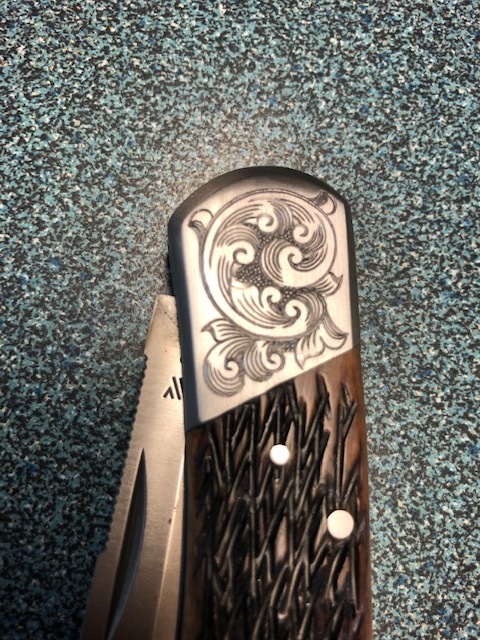This image depicts a partially folded pocket knife resting on a textured surface resembling speckled or granite stone in shades of green, black, red, and possibly blue. The knife features a brown wooden handle intricately carved with a crosshatch pattern for grip, creating the appearance of trees or branches. The carving is highlighted in black, suggesting it might be painted or filled in, and includes two small, white dots, possibly reflections. At the end of the handle is a distinctive silver cap adorned with an elaborate swirling floral motif, which resembles leaves in a swirl and bow-like design. The blade, partially visible as it is folded into the handle, is made of steel with a serrated back edge and a large notch designed for easy opening with a fingernail.